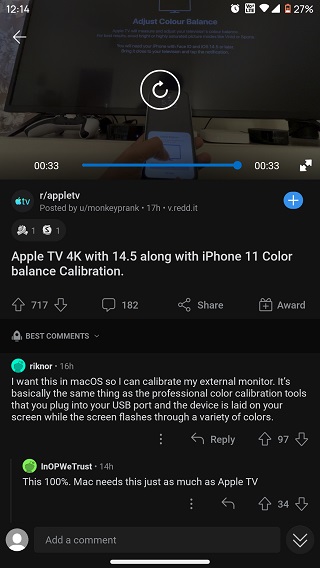This image shows a screenshot with a black background. In the upper left corner, the time is displayed as 12:14. The upper right corner features icons for the clock, Wi-Fi, and battery, which shows a charge of 27%. There is faint blue text in the center that is not legible. In the background, an image shows a person holding a cell phone in front of a computer monitor. A blue progress line beneath the image indicates that this is a 33-second video. Below this, white text on a black background reads, "R/AppleTV posted by monkeyprank 17 hours ago." The content discusses "Apple TV 4K with tvOS 14.5 along with iPhone 11 color balance calibration."